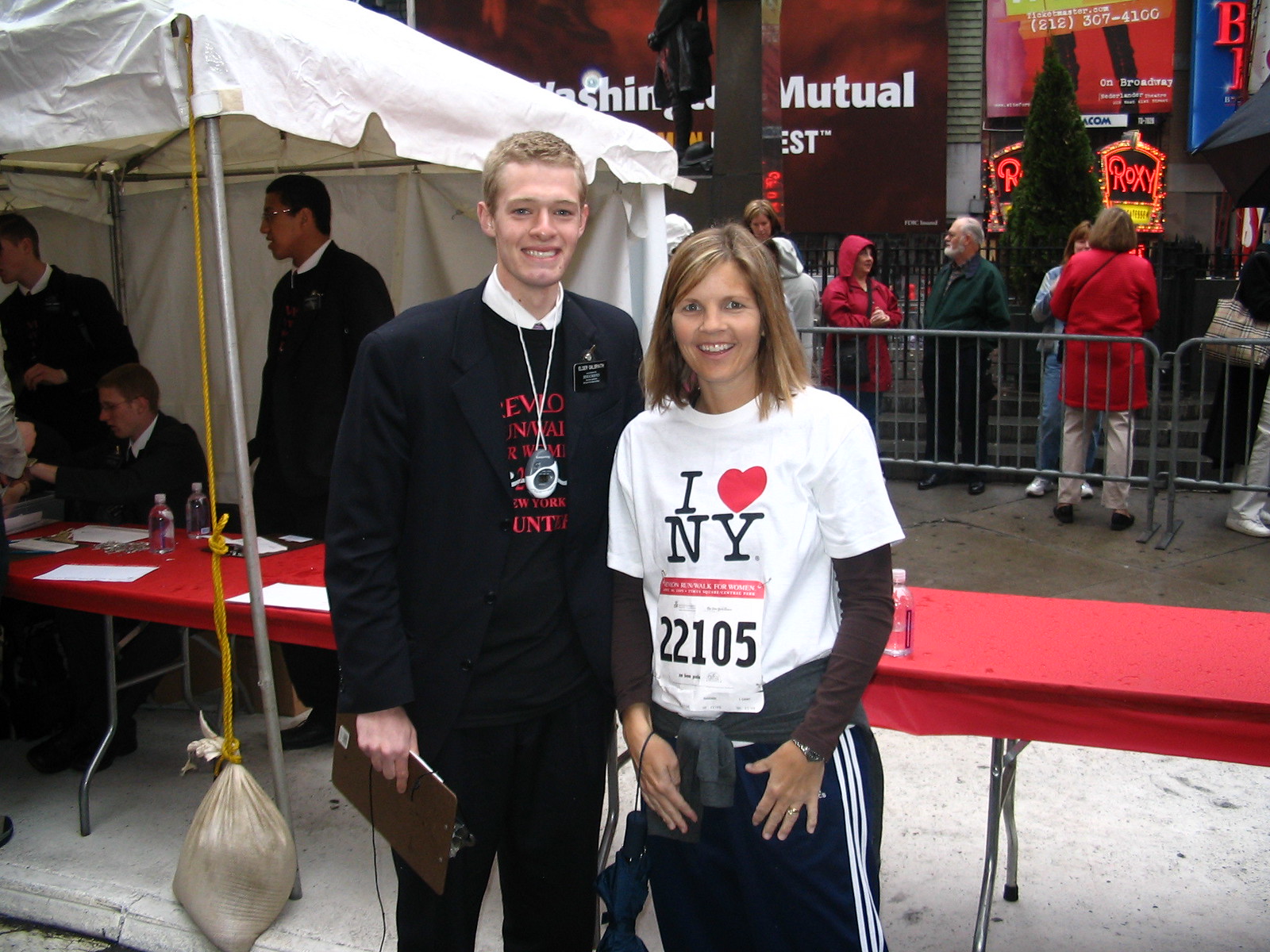The image depicts a bustling roadside event, likely a marathon or expo. At the center, two individuals are posed for the camera. The man on the left is tall and young with blonde hair, clean-shaven, and dressed in a black blazer, black t-shirt with indistinct red text, and black pants. He has a device hanging around his neck, an oval-shaped item, and a badge pinned to his blazer. He is holding a keyboard, from which wires are protruding.

To his right stands a young blonde woman wearing a white t-shirt with an "I Love New York" flyer and a registration sticker with the number 22105. Underneath, she has a brown long-sleeved shirt and is dressed in black track pants, with a jacket or sweater tied around her waist. Both individuals are looking directly at the camera.

Behind them, a long red table is visible, cluttered with water bottles and numerous papers. A makeshift tent is erected over the table on the left side of the image, inside which three men—all dressed similarly to the man in the center (black suit and white shirt)—are situated; one is seated while the other two are standing. Suspended from the tent is a large gunny bag.

In the background, billboards and large banners are visible, suggesting the setting is in a commercial area. Also seen are railings or grills, behind which a diverse group of spectators, both males, and females of various age groups, are standing and observing the event.